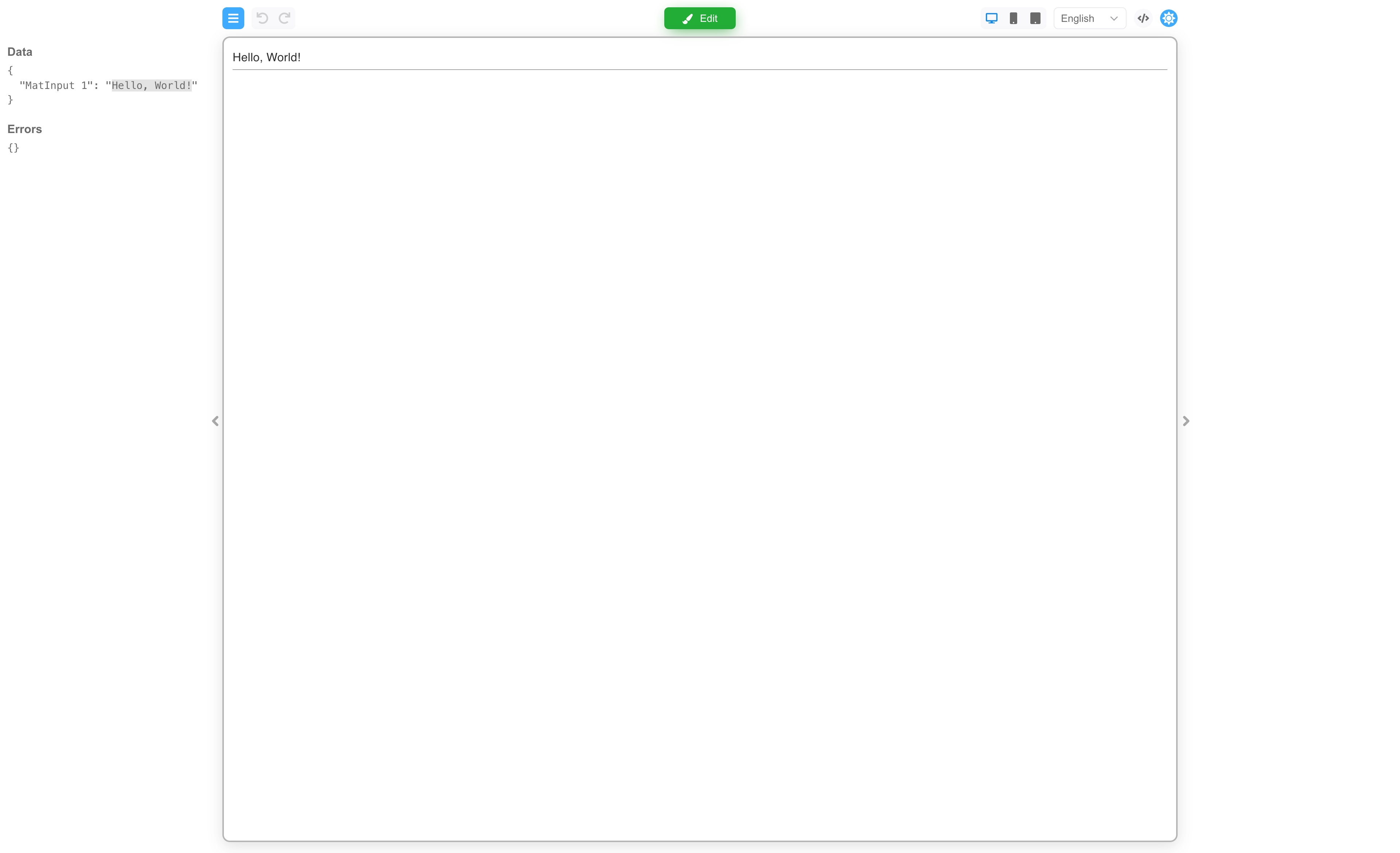The image appears to be a screenshot of a coding interface or development environment. In the upper left corner, there is a label "data", followed by a section enclosed in parentheses. This section contains the following key-value pair: `"MAT input one": "hello world"`. Next to this, there is an "errors" label accompanied by an empty array in a bracket format. 

To the right, there is a toolbar featuring several icons: a blue square with three horizontal white lines indicating a pull-down menu, a refresh button, a back arrow, and a forward arrow. 

Below this toolbar, in the center, is a green button labeled "Edit" with the word inscribed in white. Along the far right of the toolbar, there is an icon resembling a screen button, followed by two rectangular black buttons, and another pull-down menu labeled "English." Further to the right is an icon depicting a sun within a blue circle.

Beneath the main toolbar, aligned to the left, the code "hello world" is displayed under the blue pull-down menu. This appears to be both the input code and its consequent result, showing up in a specific field. This result field is outlined with a subtle gray border, forming a rectangle that is slightly longer on the horizontal axis. The clean design and clear labels suggest this image is from a user-friendly programming or data input environment, presenting the code and its output in a succinct and organized manner.